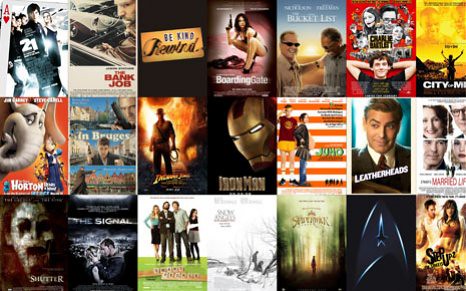The image is a computer-generated collage featuring covers of various movies positioned closely together without borders, each facing forward. The titles displayed include "21," "The Bank Job," "Horton Hears a Who," "Shutter," "The Signal," "The Birds," "Be Kind Rewind," "Boarding Gate," "Iron Man," "Indiana Jones," "Juno," "Leatherheads," "Speed," "Married Life," "Sex and the City," "Charlie Wilson's War," and "The Bucket List," among others that are difficult to decipher due to blurriness. The collage exhibits a vivid array of colors, including black, white, reddish, orange hues, and some yellow at the top right, with light blue towards the left. It envisions a total of 21 movie covers arranged in rows, forming a distinctive and vibrant advertisement for various films.